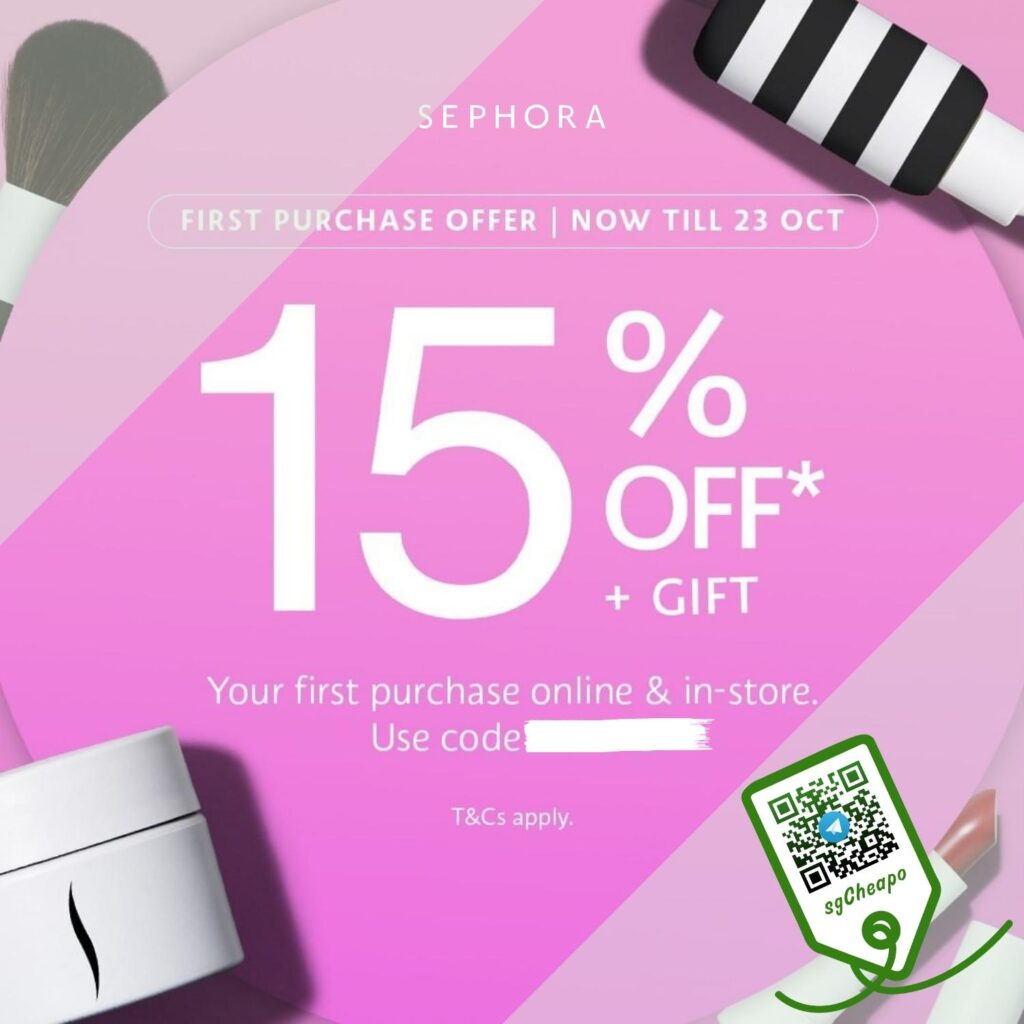This image is a promotional screen from Sephora, featuring a cosmetic-themed design with intricate details. The background is a palette of pink hues, dominated by a large, pale pink ball situated in the center, resembling a pool ball with horizontal stripes. The central stripe is a darker shade of pink, adding contrast to the composition.

In the bottom right corner, there's a green-outlined price tag that reads "SG Cheapo." Just above this, the screen advertises a Sephora first purchase offer valid until October 23. The offer includes a 15% discount and a gift with one's first purchase, applicable both online and in-store, with a blank space where a promo code would be entered. The text notes that terms and conditions apply.

On the upper right, there is a black-and-white striped image reminiscent of a Q-tip. To its left, a small, pudgy blush brush is displayed. In the bottom left corner, a white jar marked with the signature black Sephora 'S' logo is prominently featured. The overall design is visually engaging, blending promotional information with Sephora’s brand aesthetics.